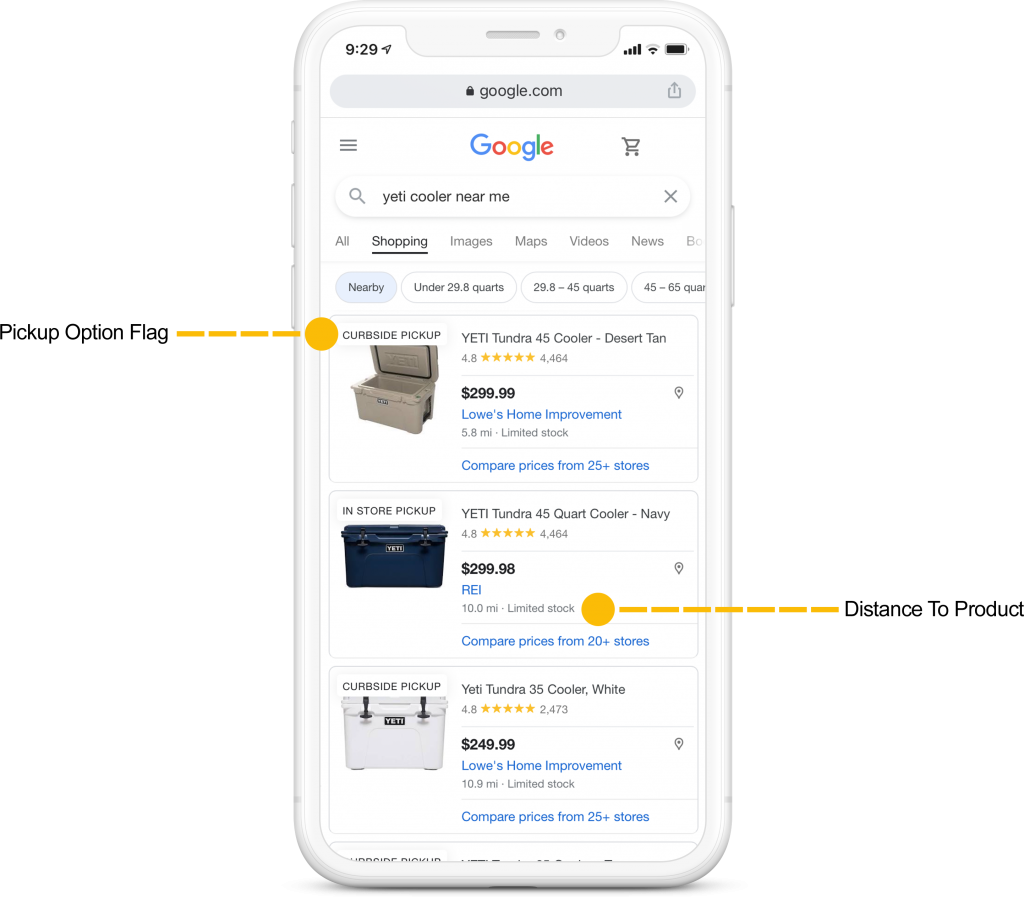The image depicts a smartphone screen with various interface elements visible. At the top of the screen, a white border houses the speaker and front-facing camera on the top left. The status bar displays the time as 9:29, a navigation arrow pointing upward and to the right, a signal icon, a Wi-Fi icon, and a battery icon.

Below the status bar, there is a long, oval-shaped search bar with a light gray background. Centered within this bar is a black padlock icon, indicating a secure connection, followed by "google.com" in black text to the right. Adjacent to the search bar on the right, there is an icon representing a share button, characterized by a square with an arrow coming out of the center. A light gray line divider separates this from a Google logo positioned further right, next to which is a shopping cart icon.

The search query "Yeti cooler near me" is displayed within another oval-shaped search bar in black text. Below the search bar, multiple search filter options are listed, including "All," "Shopping," "Images," "Maps," "Videos," and "News," with "Books" partially visible, cut off towards the right. The "Shopping" option is selected, differentiated by its black text and a bold black underline, unlike the other gray-colored options.

Further down, there are additional filter buttons in oval shapes with various labels. The "Nearby" filter is selected, indicated by its light blue background, while the rest remain white. Other filters include "Under 29.8 quarts," "29.8 to 45 quarts," and "45 to 65 quarts," with the last getting cut off towards the right.

Towards the left bottom of the screen, a "curbside pickup" label is marked by a black text flag. Four orange dashes and a large orange dot extend from the flag, pointing towards the curbside pickup label.